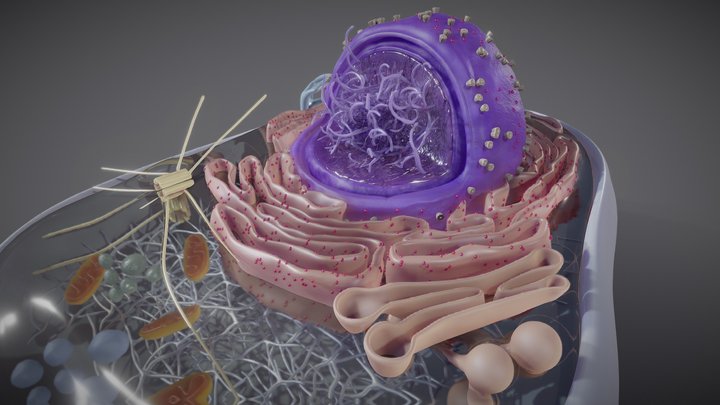The image depicts a highly detailed and complex 3D representation of a cell-like structure set against a dark grey background that fades to black at the bottom. Dominating the center is a prominent, round, purple figure that appears to be the cell's nucleus or a central organelle. This purple structure features an open section from which numerous light purple, tentacle-like filaments emerge. These filaments, which may resemble nerves or veins, are adorned with small grey or beige dots.

Encasing this central figure is a grey container or bowl-like structure, lending it a sense of enclosure. Surrounding this main structure is a series of light pink and light red, looped ribbon or tubule-like formations, reminiscent of intestines or a labyrinthine maze. These formations wrap around the purple nucleus, adding layers of intricate detail.

Additionally, there are two globular bodies positioned at the bottom right of the image, seemingly attached underneath the main structure. The image also contains various small, flat, orange, brown, and yellow globules scattered around, particularly noted in the lower left section. These could represent different components or materials within the image.

Overall, the composition gives an almost futuristic, otherworldly impression, combining abstract biological elements with a sense of organized complexity.